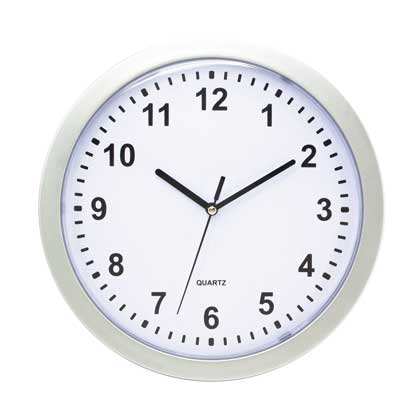This is an image of an intricately detailed clock set against a pristine, all-white background. The clock features a seamless blend of white and off-white hues, giving it a sophisticated yet minimalist appearance. The rim of the clock is a pure white, perfectly complementing the slightly off-white face, creating subtle layers of contrasting shades. The clock face is adorned with large, bold notches at each hour mark and smaller, thinner notches between them for minute increments. 

The clock's three hands are detailed with the hour hand precisely pointing at the 10, and the minute hand at the 2, indicating the time is 10:10. The second hand is positioned delicately between the 6 and 7, adding an element of dynamic movement to the still image. 

The numbers 1 through 5 are aligned on the right side of the clock face, while numbers 7 through 11 are on the left, adhering to the traditional clock layout with 12 at the top and 6 at the bottom. The sole word on the clock face is "Quartz," likely denoting the type of movement or brand, adding a touch of functional appeal to the design.

Overall, this clock, with its nuanced simplicity and precise detailing, conveys a sense of timeless elegance and reliability.